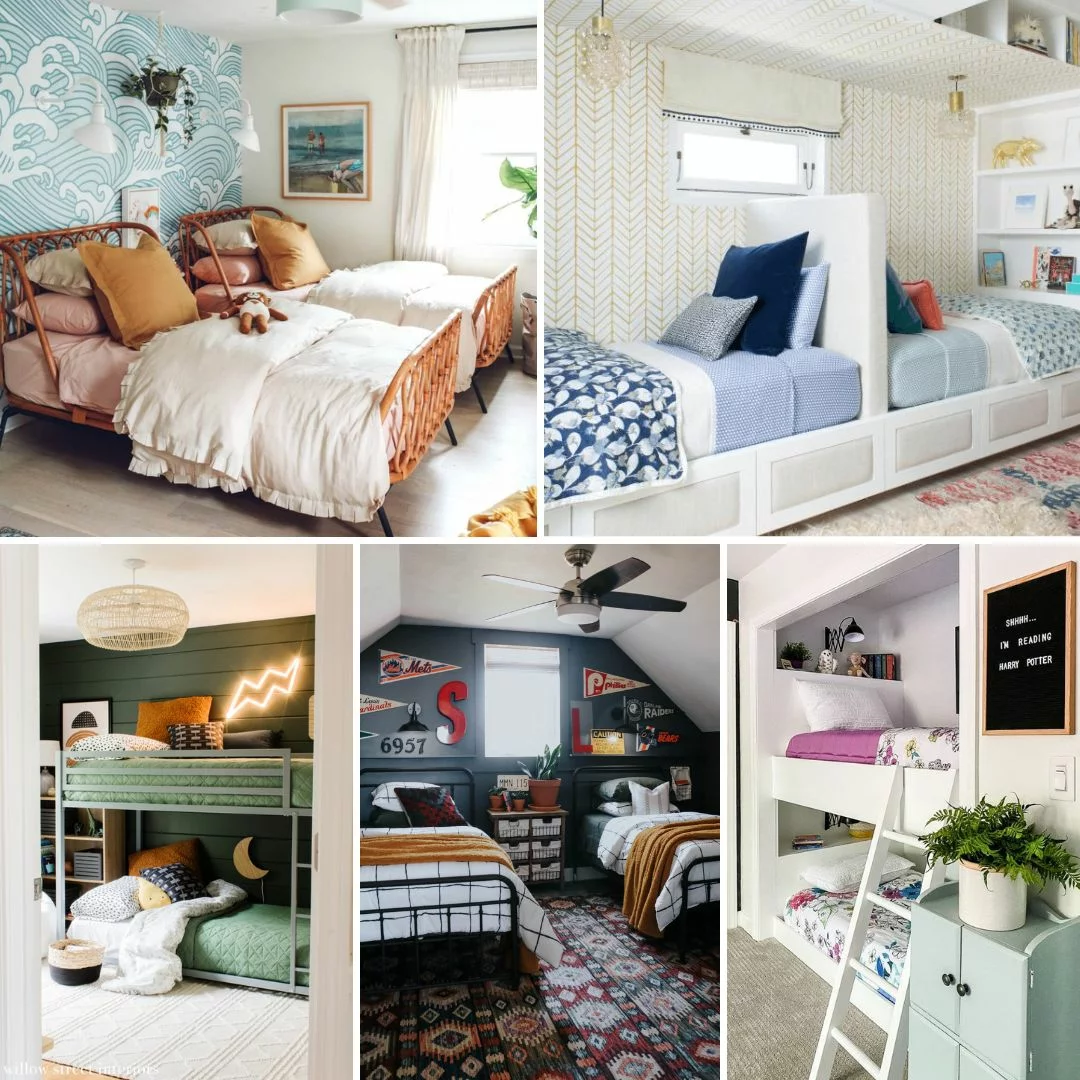This collage features five detailed images of various bedrooms. The layout consists of two images in the upper row and three in the lower row. In the upper left image, there are two twin beds with white comforters and brown pillows, including an off-white and pink pillow variant. The beds are against a backdrop of blue and green wavy wallpaper, suggesting an oceanic theme. The upper right image showcases two built-in twin beds separated by a white divider, each with drawers beneath and adorned with blue pillows and sheets.

In the lower row, the image on the left displays bunk beds with green frames and a neon lightning bolt on the wall, underlining a youthful vibe. The center lower image features two twin beds with white comforters, placed on either side of a central dresser, set against a blue wall and colorful rug. The lower right image comprises white built-in bunk beds with a matching white ladder, placed against white walls and shelving, creating a clean, integrated look.